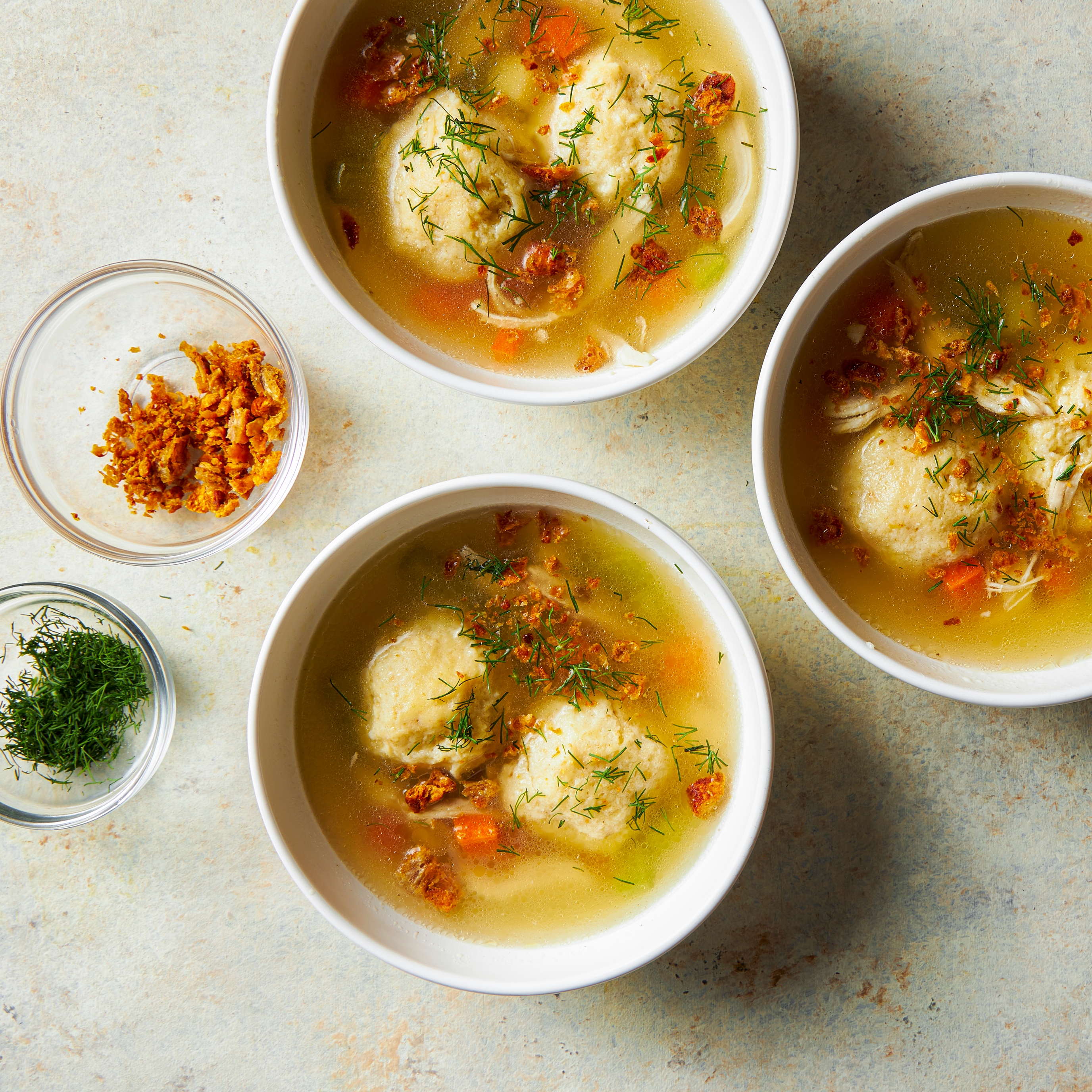The image features a close-up, top-down view of three white bowls filled with a watery, dumpling-type soup, garnished with dill leaves and other herbs. The soup also contains vegetables that could include potatoes, carrots, and leeks, adding to its rich texture and color. The bowls are set on a tiled tabletop, in a pale beige color dotted with light blue and orange flecks. Additionally, there are two smaller, clear glass dishes on the table: one holds more green dill herb leaves, and the other contains an orangish-red topping, possibly for further garnishing the soup. The entire setting rests on the pale, tiled surface, enhancing the presentation.